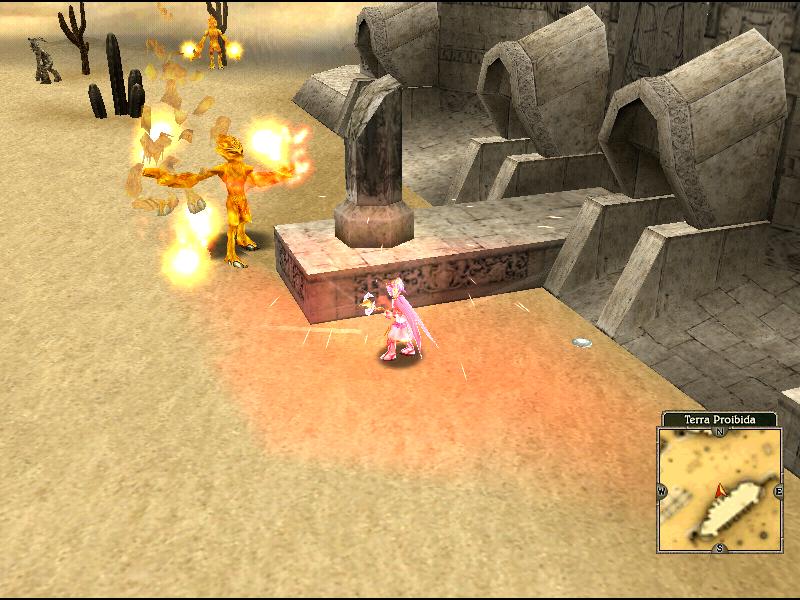The image appears to be a screen capture from an older video game, exhibiting dated, cartoonish, and anime-style graphics. The scene is set in a sandy desert area named Terra Prohibita, as indicated by a label at the top of an inset map in the lower right corner. This map also displays cardinal directions with icons and shows the player's location as a red arrow.

In the foreground, a small pink-clad humanoid figure stands adjacent to a substantial gray stone structure featuring three stone passageways and a platform extending outward. At the end of this platform stands a half-broken column with an elaborate statue.

Prominently featured is a golden, humanoid, cat-like figure emitting fiery projectiles from its hands. This fire-wielding entity stands near the stone sculpture and seems to dominate the area, which includes other figures in motion—another smaller golden figure and a more human-like character dressed in pink. The background is scattered with dark gray saguaros and additional fire-wielding figures, reinforcing the desert environment.